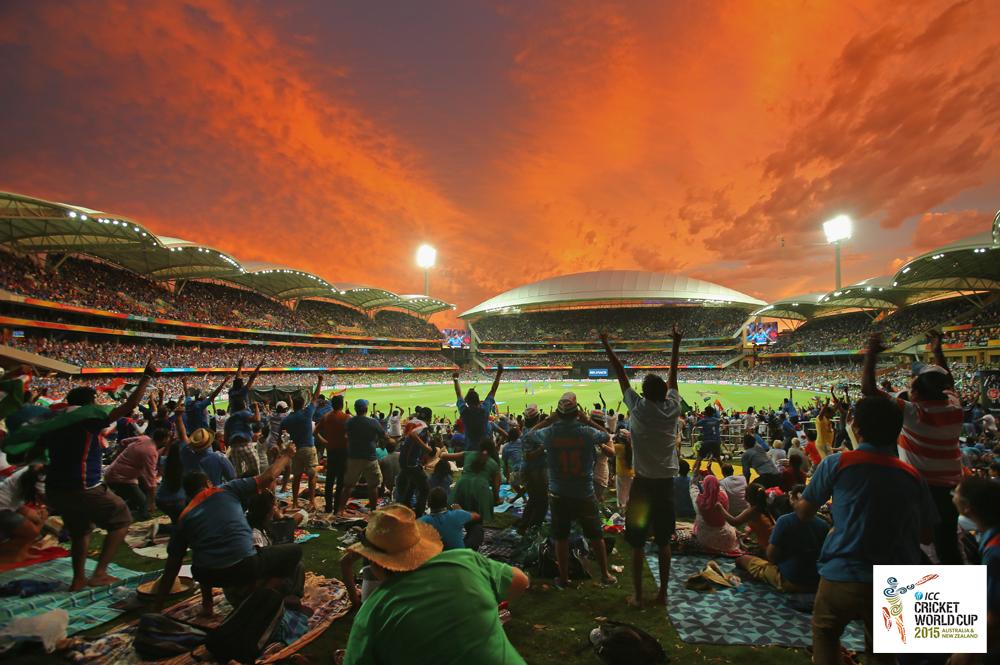This image captures the vibrant atmosphere of a jam-packed stadium during the Cricket World Cup. The stadium features a sprawling green field bordered by a multitude of cheering fans, with every seat in the tiered, spaceship-like structure taken. Overflow fans have settled on blankets and lawn chairs on the field, creating a festive, casual scene with colorful attire and raised arms in jubilation. Above the tiers, domed roofs partially cover the stands. The stadium is illuminated by lights, highlighting the orange and yellow hues of the sunset sky. Large Jumbotron screens in the corners display close-ups of the players, reinforcing the focus on the thrilling match happening on the field. Notable details include a fan in an orange cowboy hat and another in a white and red shirt, enhancing the kaleidoscope of colors and excitement as fans collectively celebrate the cricket event.